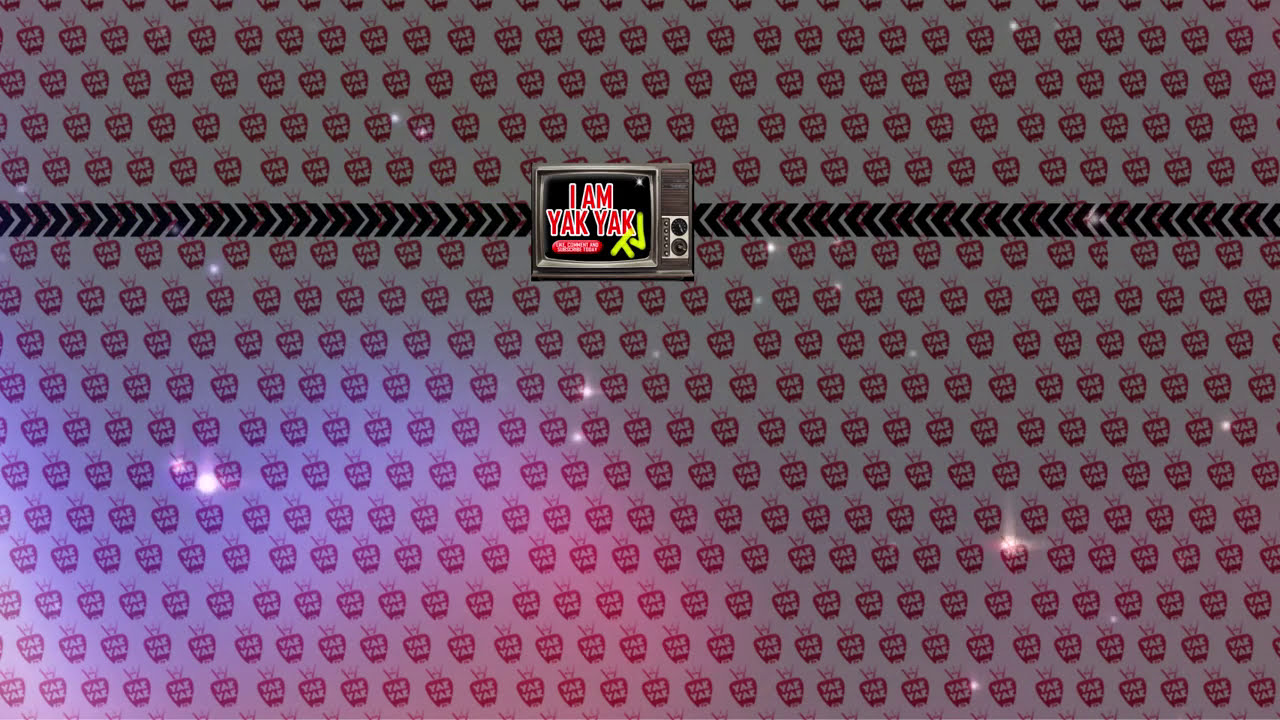The image features a white background overlaid with a detailed and repeating pattern of apple-shaped or guitar pick-like logos. Each logo is red with a tiny white text that reads "YAK YAK." These logos are arranged in diagonal rows, numbering around a hundred or more, creating a dense, visually appealing backdrop. This background pattern forms the entire backdrop of the image, lending it a rhythmic and structured look.

In the top half of the image, intersecting black arrows stretch horizontally from left to right, suggesting tire treads or a banner. These arrows converge at an old-fashioned, 70s-80s style CRT television located slightly above the center of the image. The TV has a vintage appearance, complete with dials on the front. Inside the TV screen, which is black, the text "I AM YAK YAK" is displayed in bold red, with the word "TV" written in a bright, neon yellow underneath it.

Subtle sparkles and a faint glow overlay the image, giving it a polished, slightly illuminated effect as though a light is shining down on it. In addition, there's a hint of a colorful, galaxy-like background blending softly with the white backdrop. This adds an almost otherworldly dimension with faint blues, purples, and dotted white stars, enhancing the overall visual complexity of the scene.